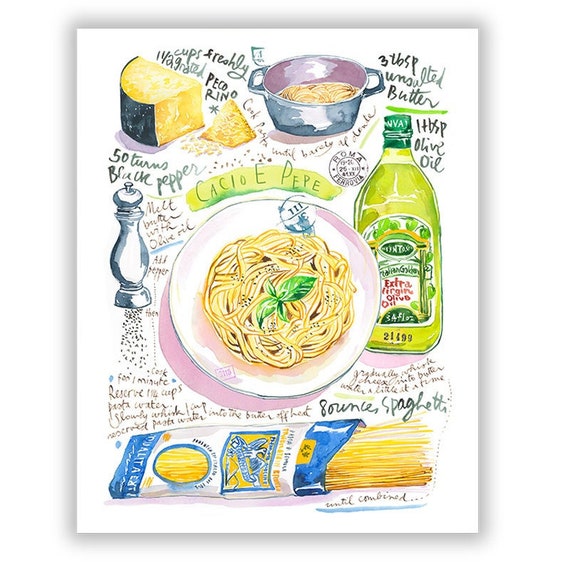This illustration serves as an artistic recipe for the dish "Cacio e Pepe," set against a white background. At the center, a lime green banner displays the dish's name, "Cacio e Pepe," in handwritten style. Below the banner sits a white plate, subtly shadowed in pink, filled with thin spaghetti noodles speckled with black pepper and garnished with a sprig of basil.

Surrounding the central plate are artistic renditions of the ingredients and tools needed for the dish. At the top left, there is a wedge sliced from a wheel of Pecorino cheese, marked as "half a cup freshly grated Pecorino." To the lower left, a silver pepper grinder is depicted, showcasing the black pepper essential for the recipe. 

To the right of the central plate, a pot containing spaghetti is illustrated, and below that, a light green bottle labeled "extra virgin olive oil" is shown. At the bottom center, an open package of dry yellow spaghetti noodles protrudes from its packaging. The entire image is framed with handwritten directions and ingredient lists, giving it the feel of a decorative sign one might purchase at a home goods store, complete with a charming and homemade touch.